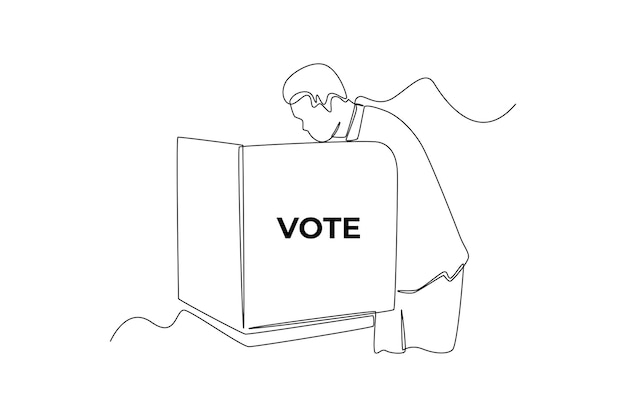This is a minimalist black line drawing of a person, likely a man with short hair, captured in a side profile as they lean over a voting booth. The image, devoid of any background details, appears to be crafted from a single, continuous line, seamlessly forming the voting booth, the person, and additional trailing lines extending from the ends of the table and the person. The booth features a partition with the word "VOTE" prominently displayed in uppercase letters on the front. The figure is simply outlined, with no intricate details, creating a stark, focused depiction of the act of voting.